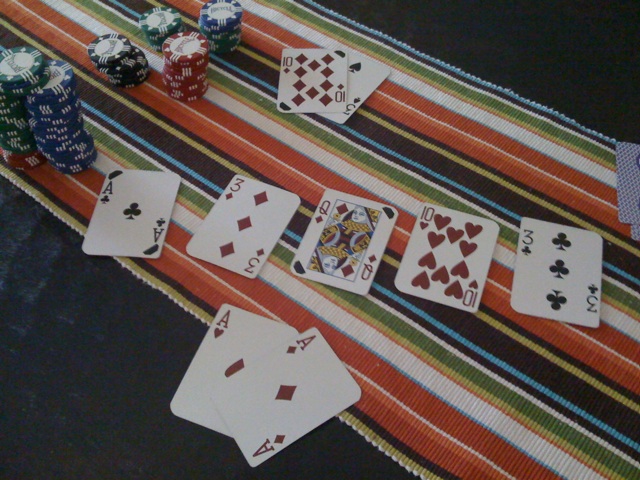This photograph captures an intense card game in progress on a large, black, solid surface. Dominating the middle of the image, from the upper left to the bottom right, is a vibrant, multicolored blanket or long tapestry. This textile, occupying about 70% of the image, features stripes in yellow, brown, orange, dark orange, white, green, and blue, creating a striking diagonal pattern.

The card game is organized into three distinct rows of cards. At the bottom center, two aces - the Ace of Hearts and the Ace of Diamonds - command attention. The middle row consists of five cards arranged from left to right: Ace of Clubs, 3 of Diamonds, 9 of Diamonds, 10 of Hearts, and 3 of Clubs. At the top center of the image, the 3 of Spades is layered beneath the 10 of Diamonds.

On the top left-hand side, there are six neatly stacked piles of poker chips, adding a competitive edge to the scene. The chips, combined with the variety of cards and the colorful backdrop, create a rich and detailed representation of the game being played.